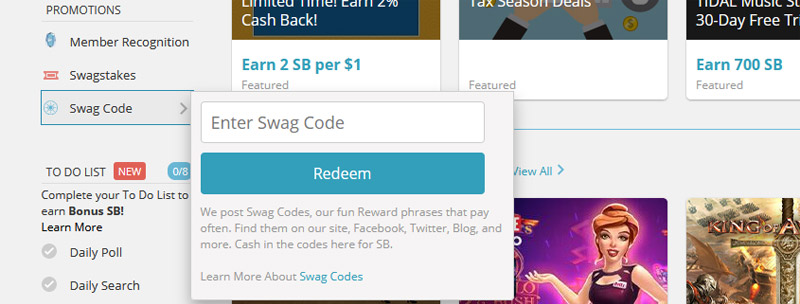This is a detailed screenshot of the Swagbucks website interface. On the left side of the screen, there's a gray sidebar featuring several options: "Promotions," "Member Recognition," "Swag States," and "Swag Code." The "Swag Code" section is expanded, revealing a pop-up menu with a search bar labeled "Enter Swag Code," a blue "Redeem" button, and a description explaining that Swag Codes are reward phrases that can be found on the site, Facebook, Twitter, blog, and more. The codes can be redeemed for SB (Swag Bucks).

Beneath this, there's a to-do list panel with tasks such as "Complete to-do list," "Earn Bonus SB," "Daily Poll," and "Daily Search." 

On the right side of the screen, various promotional icons and information are displayed. One section mentions a "Limited Time Earned 2% Cash Back," which equates to earning two Swag Bucks per dollar spent. Another section refers to a "Tax Season Deal," which doesn't specify any special rates. Additionally, there's a promotional offer for a "Title Music Service," which includes a 30-day free trial and offers an earning of 700 Swag Bucks. Despite initially appearing misleading, the 700 Swag Bucks are indeed the incentive for signing up for the $7 service rather than any trial costs.